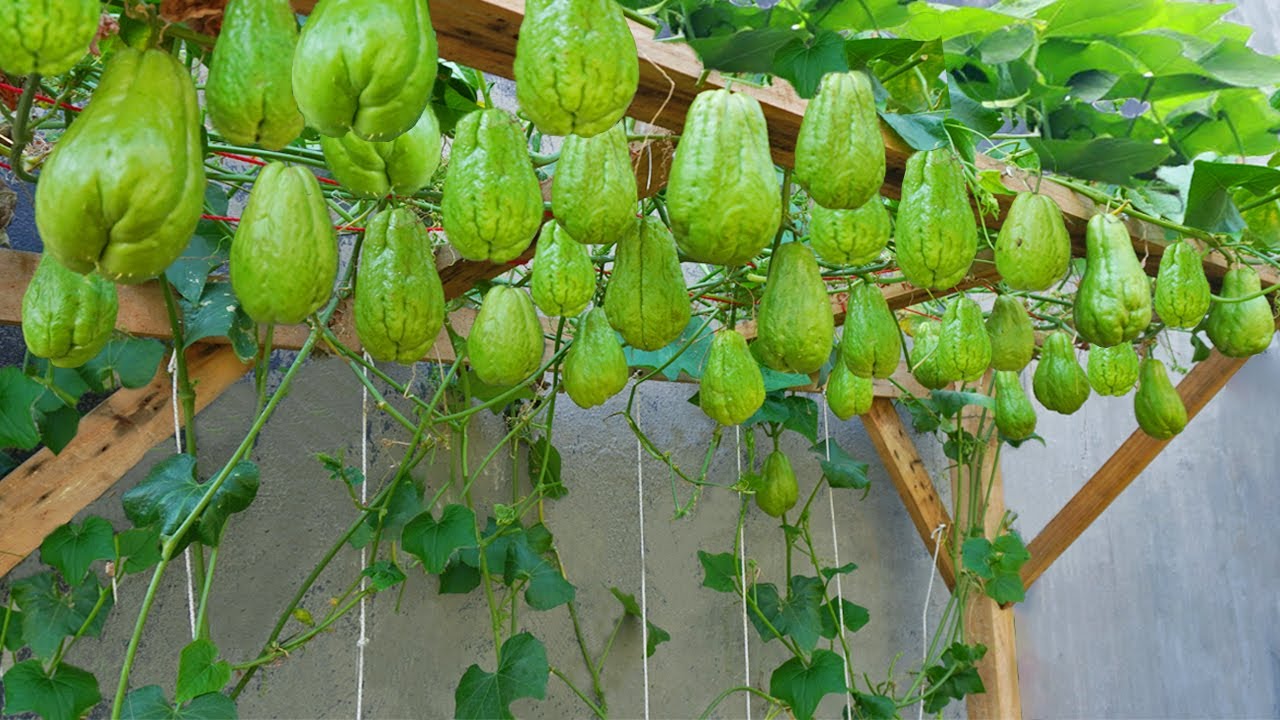This outdoor photograph captures a detailed view of a natural wooden trellis supporting a lush, green display of hanging fruits. The gray, weathered wooden wall in the background provides a rustic backdrop to the vibrant scene. The trellis structure is constructed from narrow wooden pieces forming poles and V-shaped supports, topped with large wooden slabs. Cascading down from the trellis and intertwining with white support strings are verdant vines bearing approximately 30 to 34 lime-green, pear-shaped fruits. Each fruit, measuring around 6 to 7 inches in length, exudes a fresh and ripe appearance, ready to be harvested. The green hue dominates the image, with the leaves and fruits creating a vivid contrast against the natural wood and the muted tones of the cement wall in the background. The overall scene evokes a sense of abundant, organic growth thriving within a carefully constructed and natural setting.